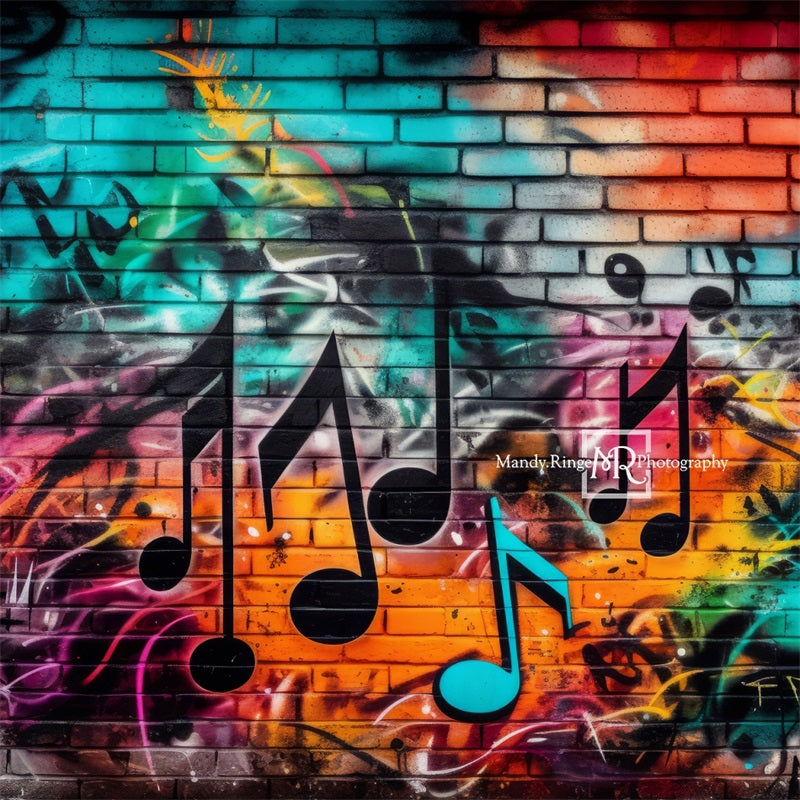The image captures a vibrant, multicolored mural painted on a brick wall, showcasing a rich palette of hues from red-orange at the top right to a bluish tint flowing toward the middle left. The middle part of the mural prominently features an array of musical notes, mostly in black, with a unique blue note near the bottom middle right. The bottom left corner transitions into a dark purple-reddish hue with textured lines of the same color, while the lower part of the mural displays stripes in white, yellow, and a cyan-turquoise gradient, particularly noticeable at the lower right. At the center, the mural bears the white text "Mandy Ring Photography" with a white square block containing the initials MR. The entire composition of the mural, filled with swirling lines and colorful designs, makes the musical notes and the text stand out vividly against the brick wall backdrop, creating a dynamic and visually engaging scene for art and music lovers alike.